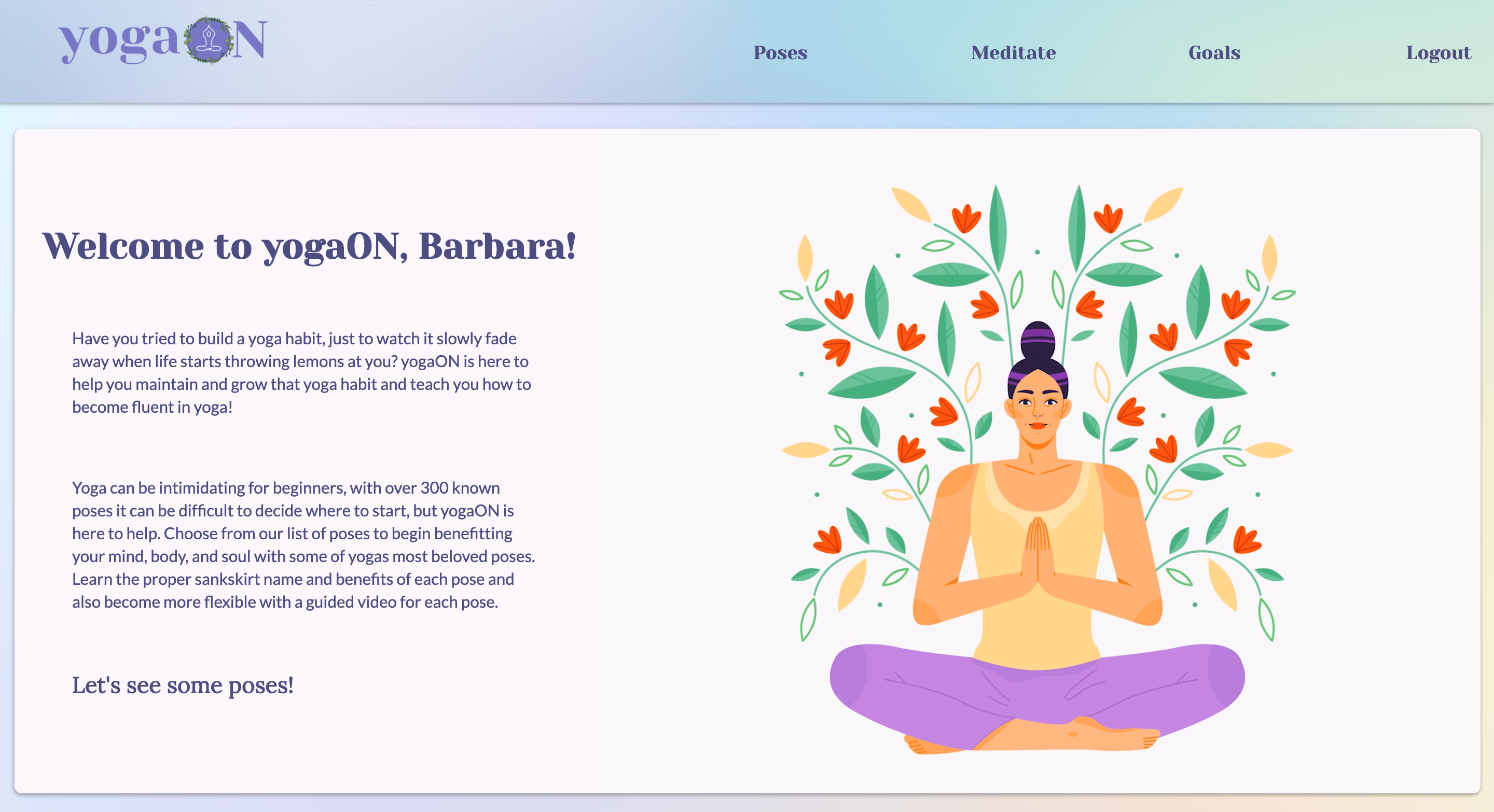**Caption:**

"This is a screenshot from the YogaOn app. At the top of the page, the app name 'YogaOn' is displayed with a unique logo where 'Yoga' is in small letters, and the 'O' in 'On' is capitalized and filled in as a distinctive symbol. The app menu across the top features options: 'Poses,' 'Meditate,' 'Goals,' and 'Logout.'

The left side of the screen presents a personalized welcome message for a user named Barbara: 'Welcome to YogaOn, Barbara.' Below this greeting, the text reads, 'Have you tried to build a yoga habit just to watch it slowly fade away when life starts throwing lemons at you? YogaOn is here to help you maintain and grow that yoga habit and teach you how to become fluent in yoga.' Additional encouraging words follow, aimed at motivating Barbara on her yoga journey.

On the right side of the screen, there is an illustration of a person, possibly a woman, sitting in a meditative pose. She's depicted sitting cross-legged with her hands in a prayer position in front of her. She wears a yellow tank top and purple pants, with no shoes. Artistic elements such as flowers, stems, and leaves surround her, symbolizing beauty, peace, and relaxation achieved through yoga."